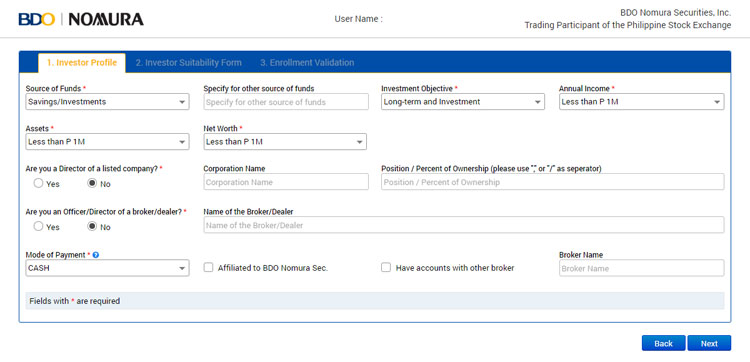**Caption:**

A detailed view of a user’s profile on BDO Nomura’s online trading platform, under the "Investor Profile" section. At the top, a blue bar spans across the page with the BDO and Nomura logos prominently displayed. Next to these logos is the user's name and the designation "BDO Nomura Securities Incorporated, trading participant of the Philippine Stock Exchange."

The first tab, marked in white with yellow letters, indicates we are viewing the "Investor Profile" section. Other tabs available include "Investor Suitability Form" and "Enrollment Validation."

Under the "Source of Funds" heading, the specified source is "Saving Investments," while other sources remain unspecified. The "Investment Objective" is set to "Long Term Investment," with an annual income, assets, and net worth all listed as less than $1,000,000.

The profile confirms the user is not a director of a listed company, with no provided corporation name, position, or ownership percentage. Furthermore, the user is not an officer or director of a broker or dealer. The selected mode of payment is noted as "cash," and it is emphasized that fields with an asterisk are required.